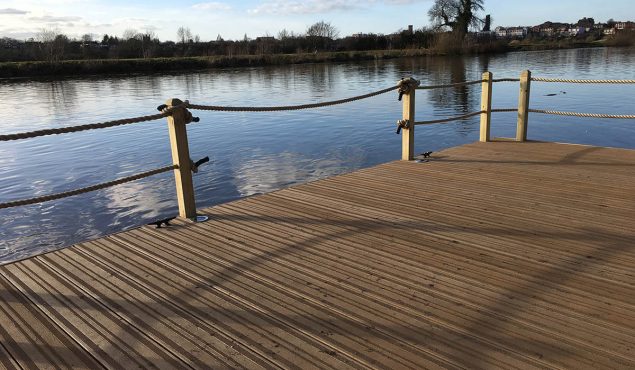The photograph captures a serene outdoor scene near a body of water, likely a pond or river, set at sunset. In the foreground, a wooden boat dock with light brown railings and posts connected by ropes (with one section missing its bottom rope) extends into the frame from the bottom and right side. The still, dark blue water stretches out in the middle, reflecting the sky and surrounding trees. In the distant background, dark brown banks are lined with trees and a few buildings, blending into the bluish-white sky with whitish-gray clouds. The reflection of the tranquil sky and trees on the water underscores the scene's peacefulness.